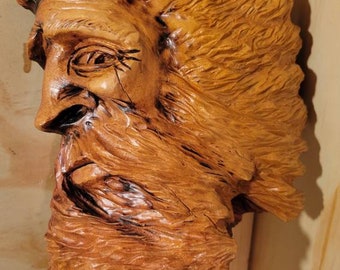This image is a detailed color photograph of a well-crafted, realistic wooden carving of a man's face, displayed in a landscape orientation. The statue, made from golden brown, honey-colored wood, exhibits rich details and delicate craftsmanship. The carving represents a man with prominent facial features, including a long mustache and a giant, flowing beard that extends into long hair, suggesting an Indian artistic influence.

The carving is shown in profile, facing the left side of the image, with the eye looking back toward the viewer. Some sections, like the eye and nostrils, are accentuated with black ink, adding definition and a lifelike quality to the piece. The wood surface includes etched wrinkles around the eye and nose, reflecting an attention to detail in representing age and character. Additionally, the faint support structure of the sculpture is partially visible beneath the chin, against a beige background that provides a subtle contrast to the wood’s warm tones.

Overall, the image captures the essence of an intricately designed statue, emphasizing the craftsmanship involved in detailed wood carving to present a historically and culturally rich representation.